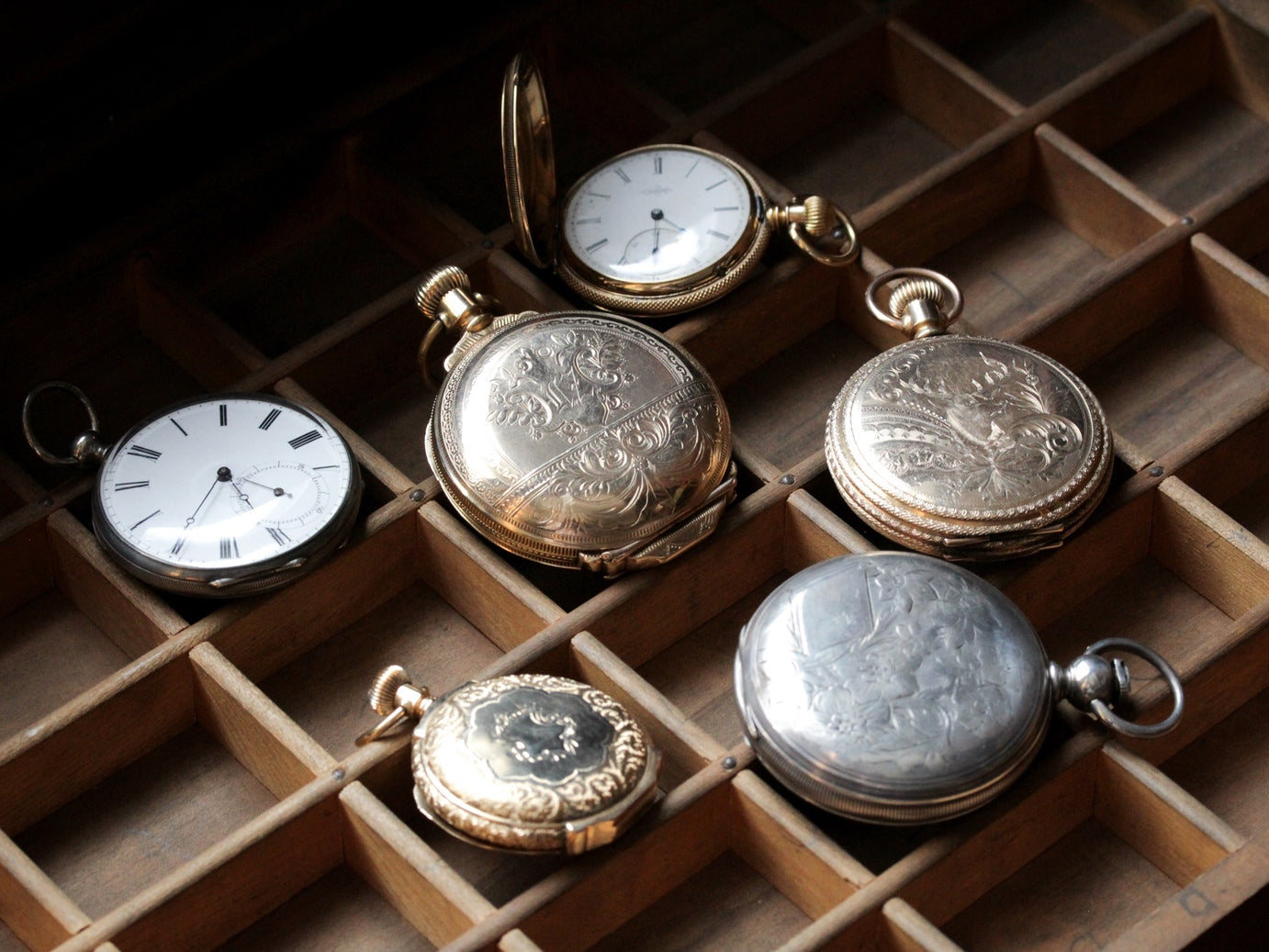In this photograph, a collection of six pocket watches is meticulously arranged atop an antique wood printer's box. This box, historically used to organize tiny letterpress blocks in its numerous small compartments, offers a rich backdrop of dark brown and gray wood tones. The pocket watches vary in design and detail. Two of them—situated on the upper left and right—have open faces displaying white dials with black Roman numerals. One is a gold pocket watch with an open lid, and the other lacks a lid entirely. The remaining four watches, all in metallic hues ranging from gold to silver, feature intricately engraved lids. These engravings include a floral design, an elk or deer motif, ornate borders with smaller floral circles, and faded leaf patterns on the silver-white watch in the foreground. Although intended for smaller objects, the compartments of the printer's box offer a unique and nostalgic setting for these elegant timepieces.